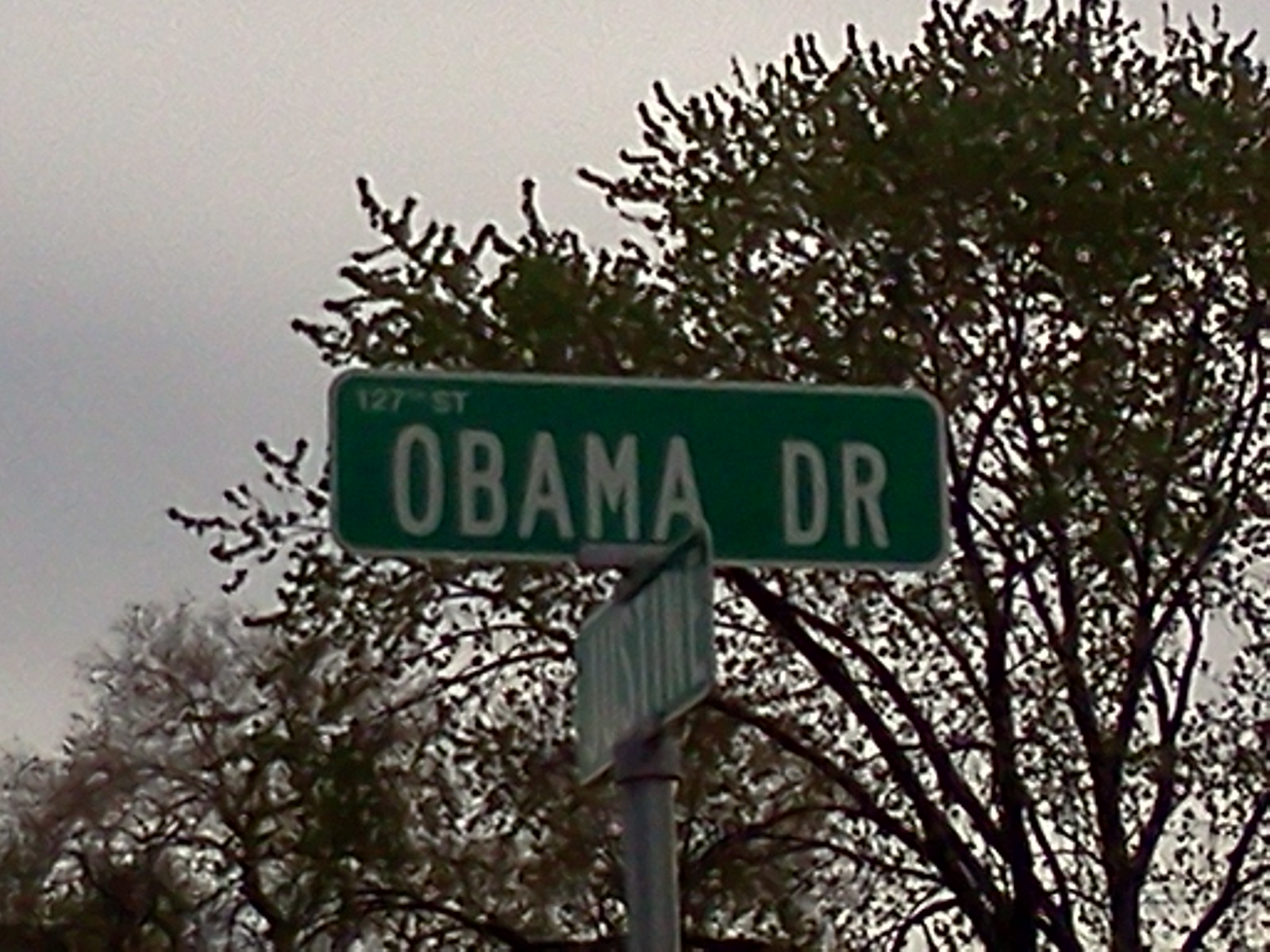Close-up of a street sign at the intersection of Obama Drive and 127th Street. The green street signs with white borders and white lettering indicate the corner crossing of the two streets. The sign for Obama Drive is prominently displayed, while another sign below it, facing a different direction, marks Justine Street. Both signs are mounted on a metal pole. In the background, the sparse tops of trees with few leaves are visible, silhouetted against an overcast evening sky, adding a moody ambiance to the scene.